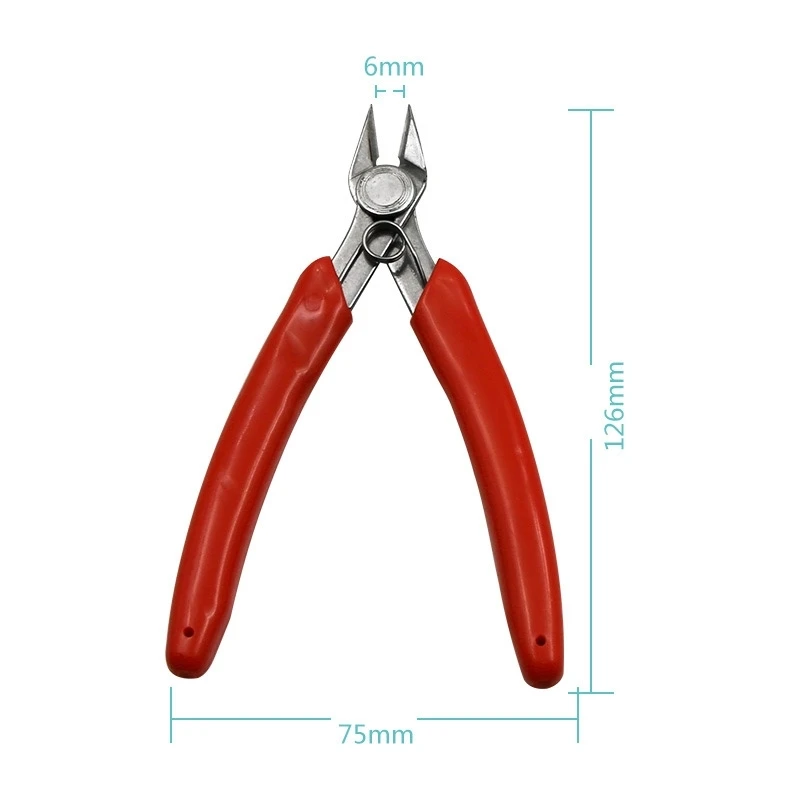The image features a detailed close-up of sturdy, silver-colored wire cutting scissors with sharp, beveled cutting edges specifically designed for precision. These small but durable cutters, measuring 126 millimeters in height and 75 millimeters in width at their widest point, are fitted with ergonomic handles for comfortable use, wrapped in a vibrant red, slightly rubbery plastic material. The handles also feature two small hollowed-out holes, possibly for hanging storage. The sharp beveled cutters, spaced 6 millimeters apart, make these tools ideal for snipping delicate wires, small metal pieces, string, or even thin wood. The combination of robust construction and the ergonomic design of the red handles underscores their utility and longevity as a practical hand tool.